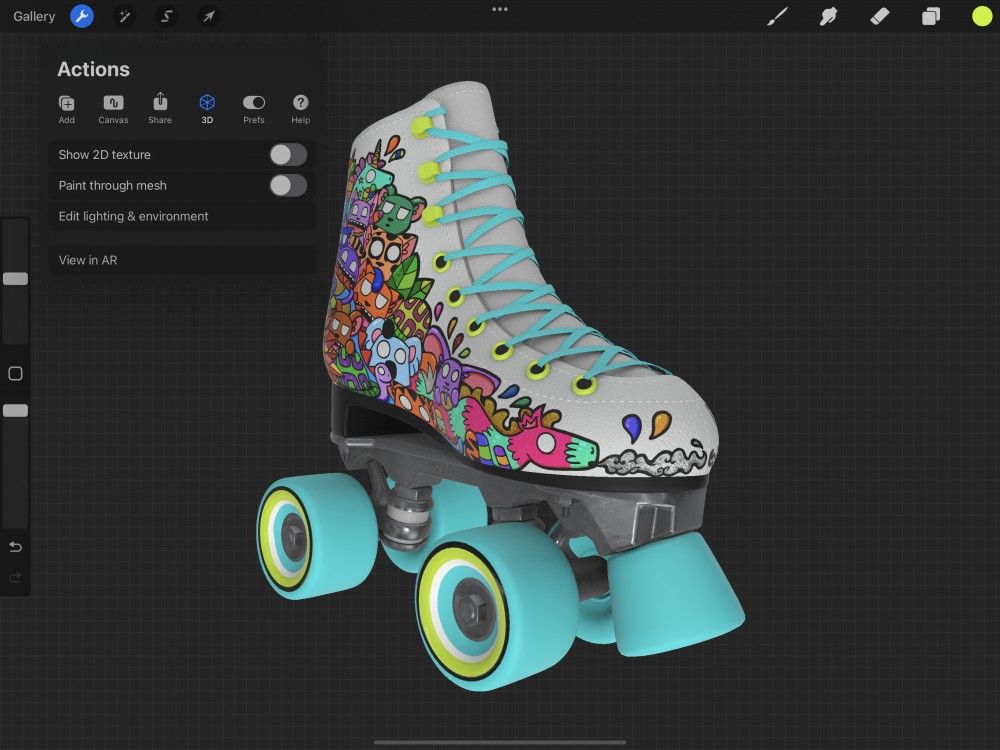This image displays a detailed 3D rendering of a roller skate within a sophisticated 3D image generation interface, possibly resembling an AutoCAD system, set against a gray background grid. The interface is populated with various settings and tools, including a top menu bar featuring icons for gallery, a wrench, a pen, an 'S', and a cursor, and a side menu with a paintbrush, an unidentified object, a pipe wrench, an eraser, a multi-page icon, and a circle. The primary display is split into multiple sections, with the upper left corner highlighting options such as 'Actions', 'Add', 'Canvas', 'Share', '3D' (currently selected), 'Press', and 'Help'. The 3D tab includes sub-options for 'Show 2D Texture', 'Paint Through Mesh', 'Edit Lighting and Environment', and 'View in AR', though the toggles for 'Show 2D Texture' and 'Paint Through Mesh' are off.

Central in the image, atop the grid, is an intricately detailed roller skate, characterized by a white shoe adorned with vibrant, cartoon-style graffiti featuring a range of animals such as a dragon, dogs, a bat, a cat, a turtle, and a bear, rendered in lively hues of blue, pink, red, purple, yellow, orange, and green. The shoe is equipped with blue laces threaded through yellow eyelets and hooks, and the metal underside, which supports the shoe, appears gray, white, and black. The skate is held together by a dark gray frame and features blue wheels with yellow, black, and white details on the inside hubs, as well as a blue rubber stopper pad at the front.